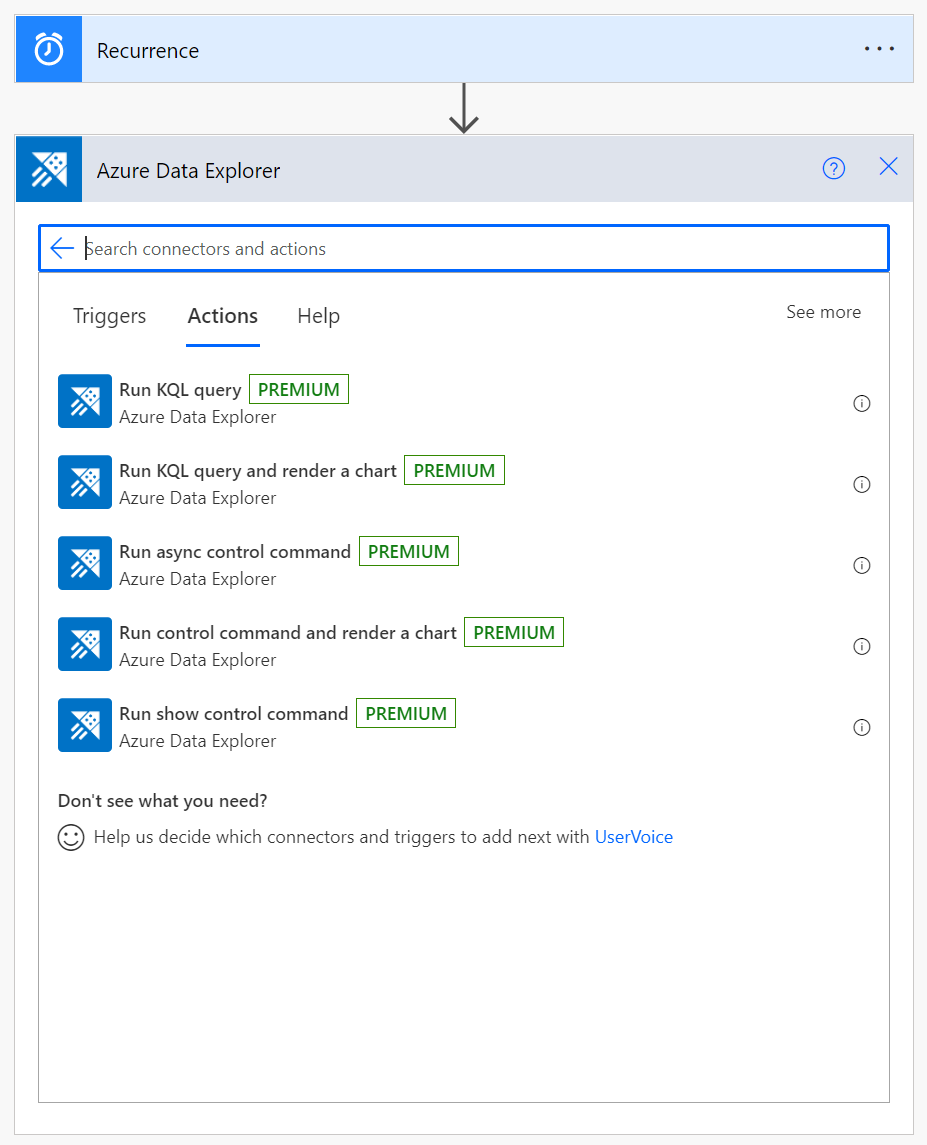The image displays a webpage sectioned into two interactive panels that seem to be designed for a technical or software-related workflow. 

The upper panel is titled "Recurrence" and is marked with an alarm clock icon, suggesting that this section is centered around recurring tasks or scheduled actions. An arrow points downward from this panel to another section labeled "Azure Data Explorer," which is indicated with a paper airplane icon, hinting at a connection or data exploration functionality within Microsoft Azure.

Further down, there's a search bar labeled "search connectors and actions," allowing users to find specific functionalities. Below this search bar, a list of available actions is displayed:

1. Run KQL query
2. Run KQL query and render a chart
3. Run async control command
4. Run control command and render a chart
5. Run control command
6. Run show control command

Each of these actions has a "premium" tag next to it, indicating that they are part of a premium subscription plan.

The bottom of the interface includes a prompt: "Don't see what you need? Help us decide which connectors and triggers to add with user voice." This suggests that users can contribute feedback to improve or expand the service's capabilities.

Overall, the image appears to be a configuration interface for automating tasks and queries within a technical platform, likely offering advanced data handling and exploration functionalities.